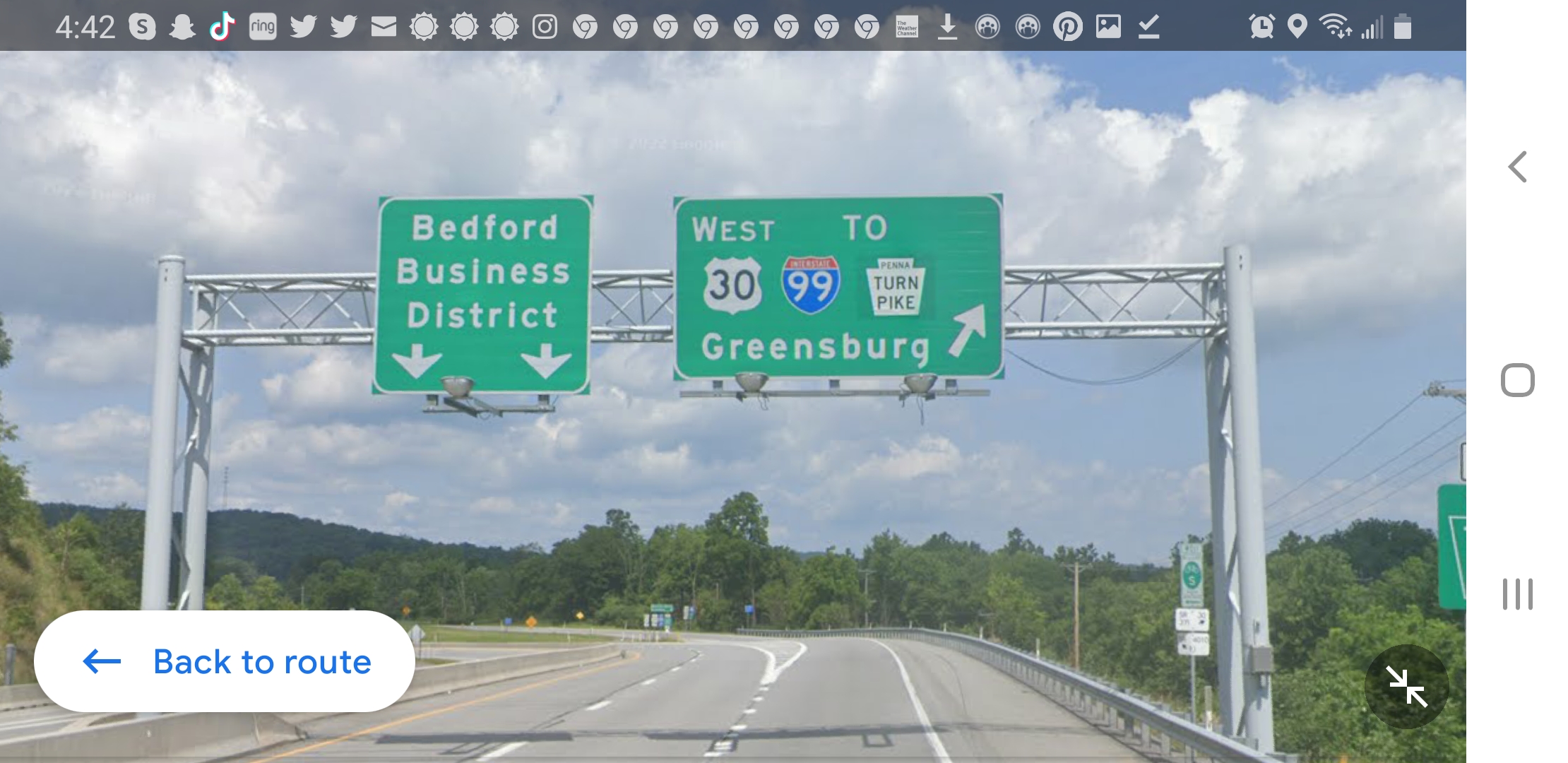The image is a detailed screenshot of a Google Maps Street View from a computer desktop, giving the impression of driving down a six-lane highway. Visible at the top is a black bar displaying the time as 4:42 alongside numerous icons, including open tabs and various programs like TikTok, Twitter, Google Chrome, and Skype. A Wi-Fi signal icon is also present to the far right. The central focus is on a white steel beam structure spanning the highway with two green highway signs. The left sign, guiding traffic into the Bedford Business District, directs drivers into the left lanes. The right sign, indicating directions west to Greensburg along Route 30, Interstate 99, and the Turnpike, points to the right lanes. The backdrop features a green tree line with dark green hills extending across the horizon, contributing to the natural scenery. Additional interface elements include a "Back to Route" button at the bottom left, suggesting navigation options, and symbols suggesting the display might also be accessible on a mobile device.